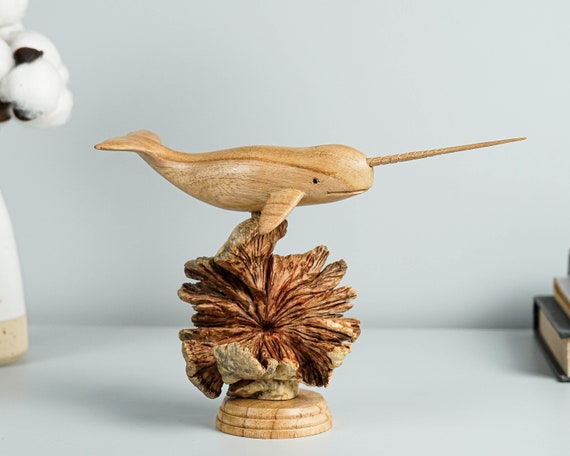This photograph features a detailed wooden sculpture of a narwhal, a marine mammal known for its distinctive long horn protruding from its forehead. The narwhal, depicted in a beige-colored wood finish, is intricately carved and rests on a wood base shaped to resemble sea coral or possibly a flower, complete with segmented, petal-like designs. The base itself resembles three stacked discs with horizontal lines, giving it a tiered appearance. To the left side of the image, there's a partially visible white vase filled with cotton-like flowers, while to the right, there is a stack of books. The background of the shelf is white, complementing the granite-like material of the shelf itself, making the sculpture a striking decorative piece.